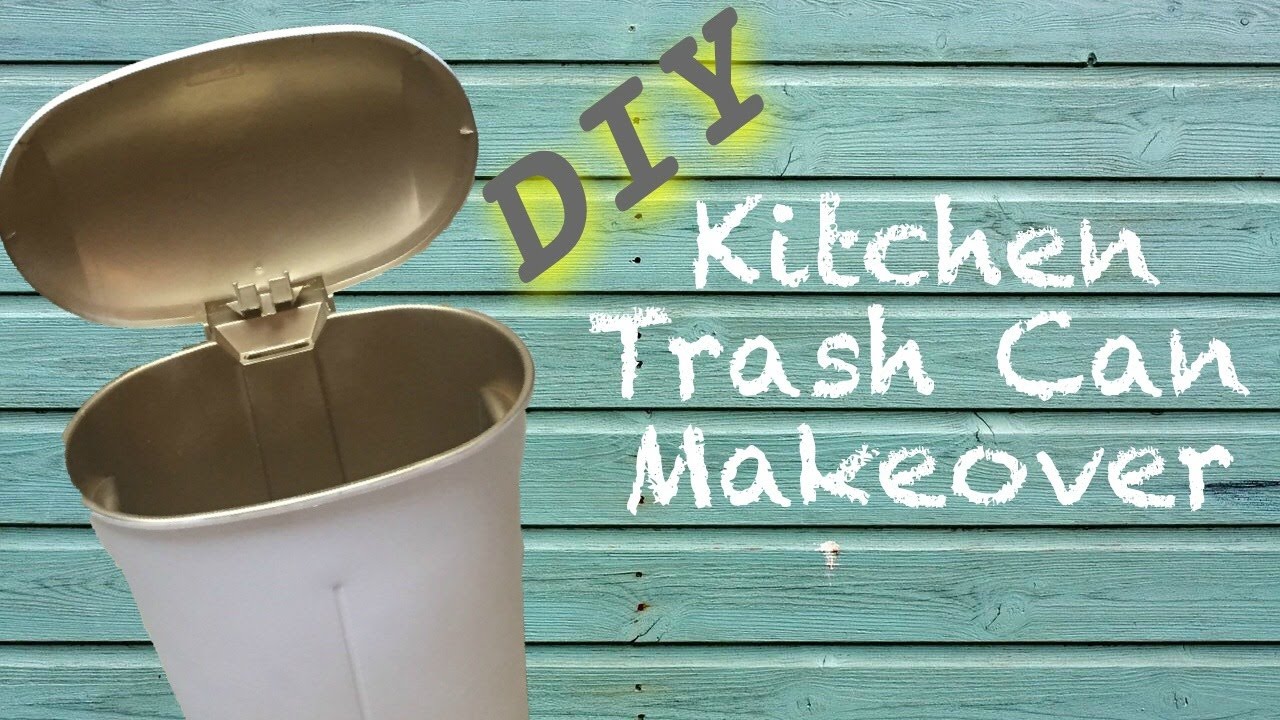This advertisement, presented in a rectangular, landscape layout, features the word "DIY" prominently in gray font with a distinctive yellow shadow. On the right-hand side, it declares "Kitchen Trash Can Makeover" in elegant white text set against a backdrop of horizontally aligned, light blue wooden planks. On the left side of the advertisement, there is a detailed photo of a trash can with its lid open, revealing a chrome-colored interior. The trash can is white on the outside, tilted slightly to the left and angled upwards, giving a clear view of its design and functionality.